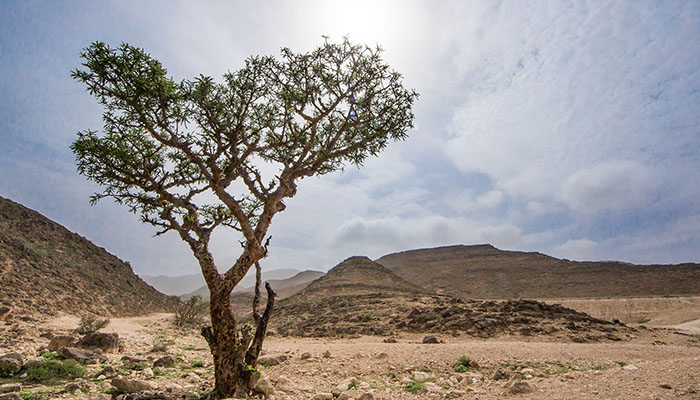This photograph captures an arid desert landscape under a partly cloudy sky, with the sun peeking through wisps of white clouds. The sky, which occupies roughly the top half of the image, has a light blue hue softened by the clouds. Below the sky, the terrain is mostly dry and barren, dominated by shades of brown and beige, with an occasional hint of green vegetation.

In the background, the horizon features a series of gray-brown, mesa-like mountains and hills, with a distinct triangular peak near the center of the image. The foreground, contrasting sharply with the expansive sky and distant hills, features a mix of sand, dirt, small pebbles, and sparse scrubby plants.

A prominent feature of the foreground is a gnarly tree, situated just off-center to the right. This tree has a sturdy brown trunk that forks into a Y shape and extends into multiple branches with spindly green leaves at the top, providing a stark contrast to the otherwise stark environment. Additional small patches of dry, scrubby vegetation are scattered across the scene, particularly noticeable in the right corner and the slope on the left.

Overall, the photograph portrays a desolate yet striking desert scene, with the rugged tree serving as a focal point amidst the expansive, dry landscape and the vast, cloud-dotted sky overhead.